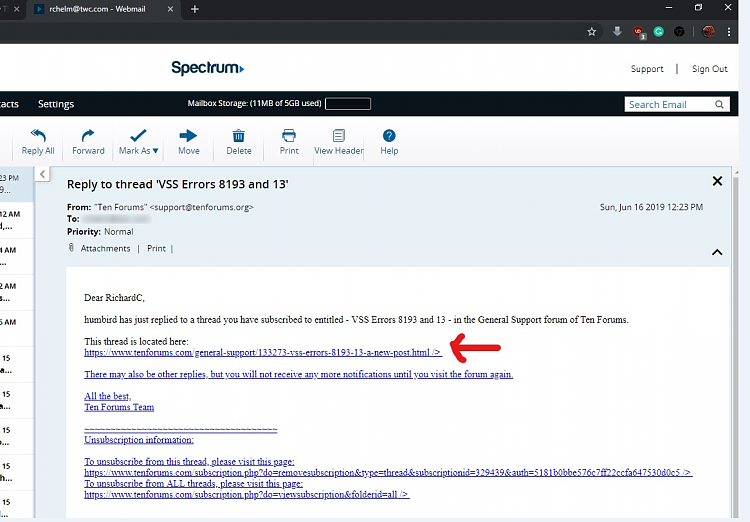The image depicts a detailed view of a webmail interface hosted on tvc.com. At the top, there is a black header displaying the current time along with links to TVC's webmail platform. Directly below, a search bar stretches across the screen, providing a space for users to type queries.

Beneath the search bar, there is a white background section displaying the Spectrum logo in blue, accompanied by a blue right arrow. Also present are options for "Support," "Align," and "Sign Out." Following this section, a black box contains options for "Settings" and "Mailbox Storage," indicating that 11 megabytes of the available 5 gigabytes have been used. Inside this box, there's a small white square with a black center.

Adjacent to these elements is another search box labeled "Search Email." Below it, light blue buttons offer various functionalities including "Reply All," "Forward," "Mark as," "Move," "Delete," "Print," "View Header," and "Help." Partial views of additional interface elements are visible on the left side of the screen.

On the right, there's a prominent blue box containing a message. The subject line reads "Reply to thread VSS errors 8193 and 13." The message originates from 10forums, sent by support@10forums.org, with the recipient's address obscured for privacy. The email is marked with normal priority, and mentions attachments and printing options. The body of the message addresses Richard C., informing him about an update on a subscribed thread regarding VSS errors 8193 in the General Support Forum of 10 Forums. A large red arrow points to a hyperlinked address, presumably leading to the thread.

The message is set against a white background within the blue box, with a close ('X') button at the top right corner. The timestamp reads "Sunday, June 16, 2019, 12:23 PM," and there is an "up" arrow option visible at the top-right corner as well.